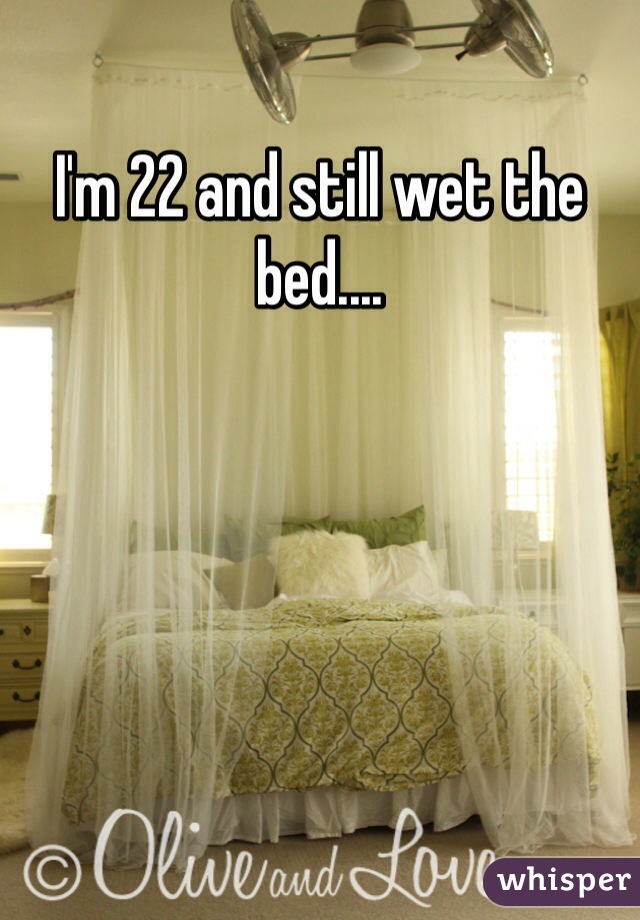The image depicts a well-arranged bedroom centered around a large bed, possibly king-size, adorned with a greenish comforter. The bed is prominently positioned in the middle, surrounded by a sheer, white canopy-like curtain that hangs from curved rods secured to the ceiling. The curtains are translucent and frame the bed, leaving an opening at the front for easy access. 

Above the bed, in white superimposed text, the image reads, "I'm 22 and still wet the bed." At the bottom, it features a trademark or copyright notice with the name "Olive and Love," followed by the word "Whisper," indicating that this image is sourced from the Whisper app or website.

The bedroom's color palette includes shades of black, white, silver, gray, various greens, tans, yellows, some off-white, and a bit of blue. The bed is accessorized with white furry pillows and additional green pillows. Surrounding the bed, one can see some decorative elements such as plants and furniture, including a bureau on the left side beneath an open or uncovered window, and another window on the right side. The floor is carpeted, enhancing the cozy ambiance of the room.